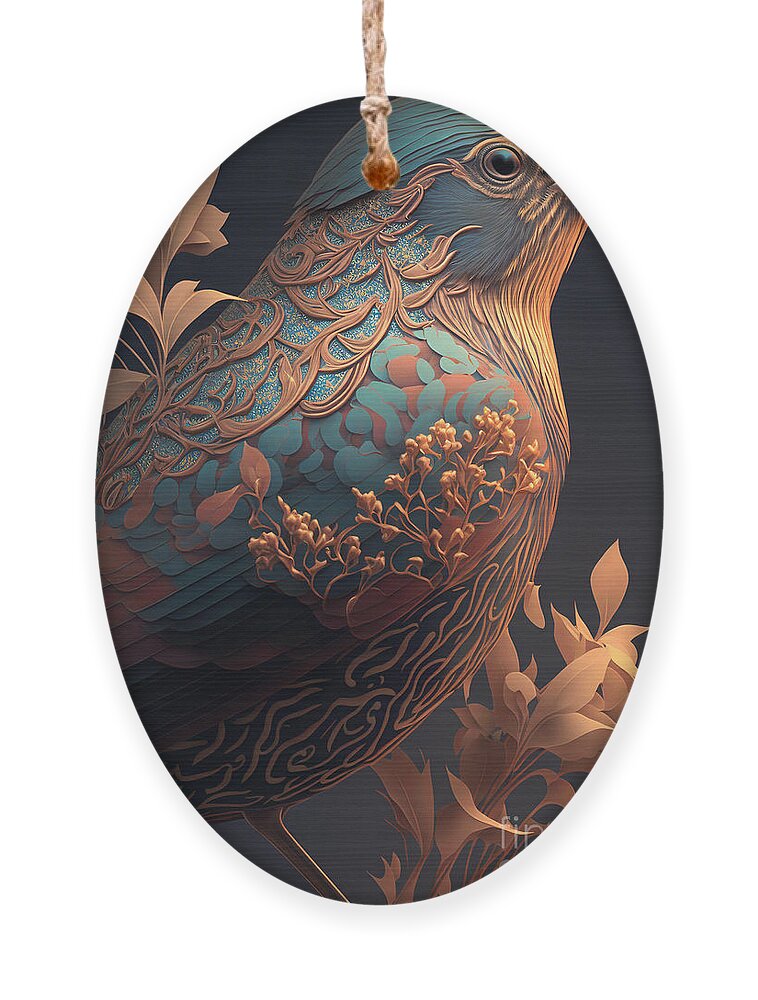This image showcases an oval painting, possibly a print, displayed against a charcoal black background. The artwork is suspended, resembling an ornament, with a thin, short string attached at the top, ending in a red dot where it meets the piece. The painting features a partial profile of an ornate bird, predominantly painted in muted dark blue with goldish and reddish accents. The bird's chest and back are adorned with intricate designs, including interlocking vines and worm-like structures, all rendered in a copper-like hue. Striated copper feathers cover the bird's throat, and bushes and rocks, also in copper, emerge where the wing joins the breast. The bird's head is turquoise, with a turquoise eye resembling a peacock's color. Surrounding the bird are groupings of brown leaves and stems, positioned at both the top left and the far bottom right of the painting. Only a portion of the bird is visible; the beak, lower body, and tail are missing, and just one leg, painted brown, is shown.